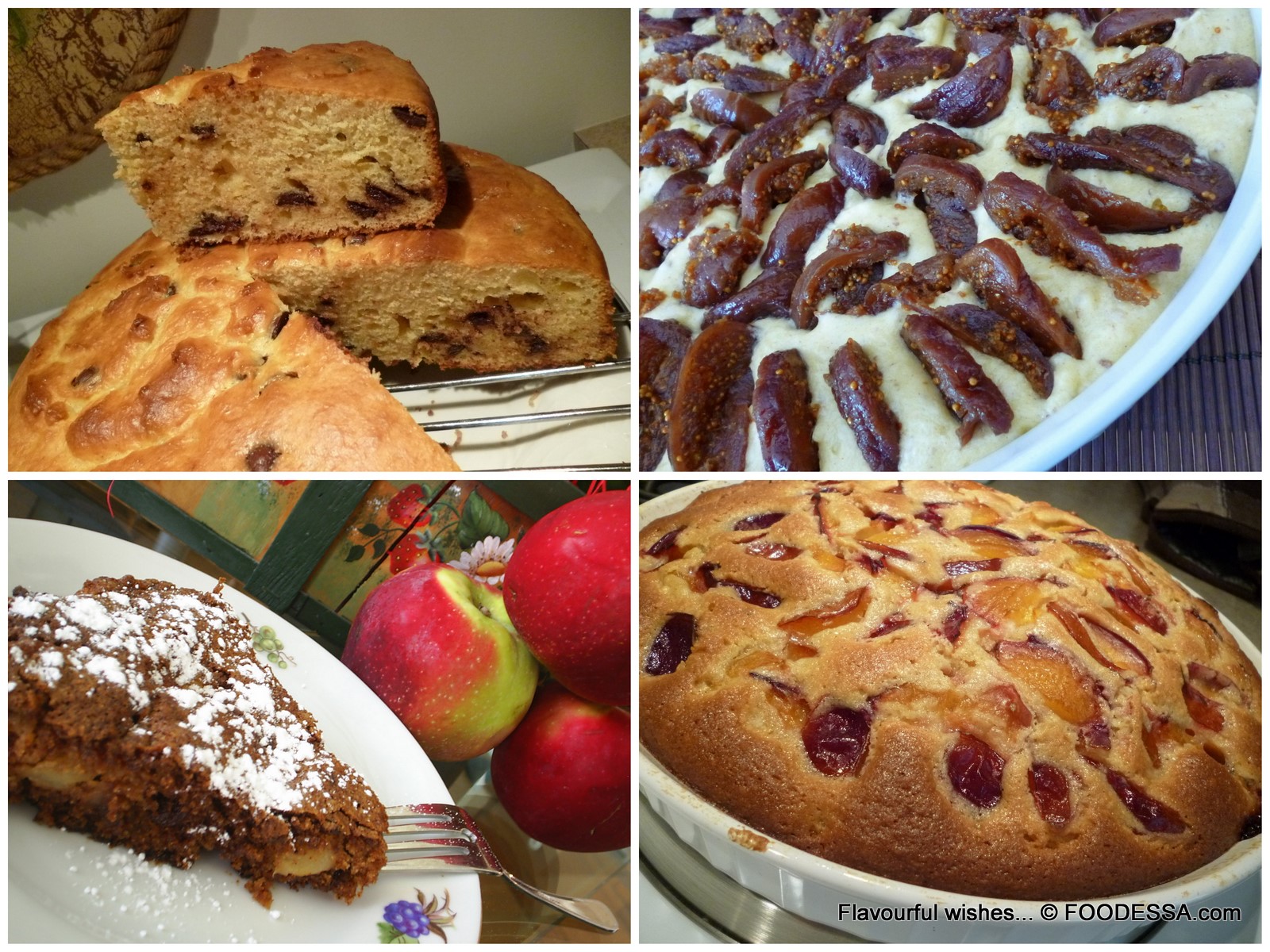This image features a quad of four food pictures, each occupying an equal-sized square. The top left square showcases a round, cake-like item with a wedge cut out and propped on top. The cake has a light brown dough and appears to contain raisins or fruit baked inside. Moving to the upper right, there's a dish with a creamy, white texture, topped with halved dates or a similar brown item. The lower left square presents a slice of strudel or pie with a brown, crumbly dough, dusted with powdered sugar, on a white plate adorned with a painted blackberry and accompanied by three red apples with green leaves and a silver fork. Finally, the lower right square features another round, fruit-studded cake on a white dish, similar to the top left item. The bottom of the image reads "Flavorful Wishes," with a copyright to foodessa.com.